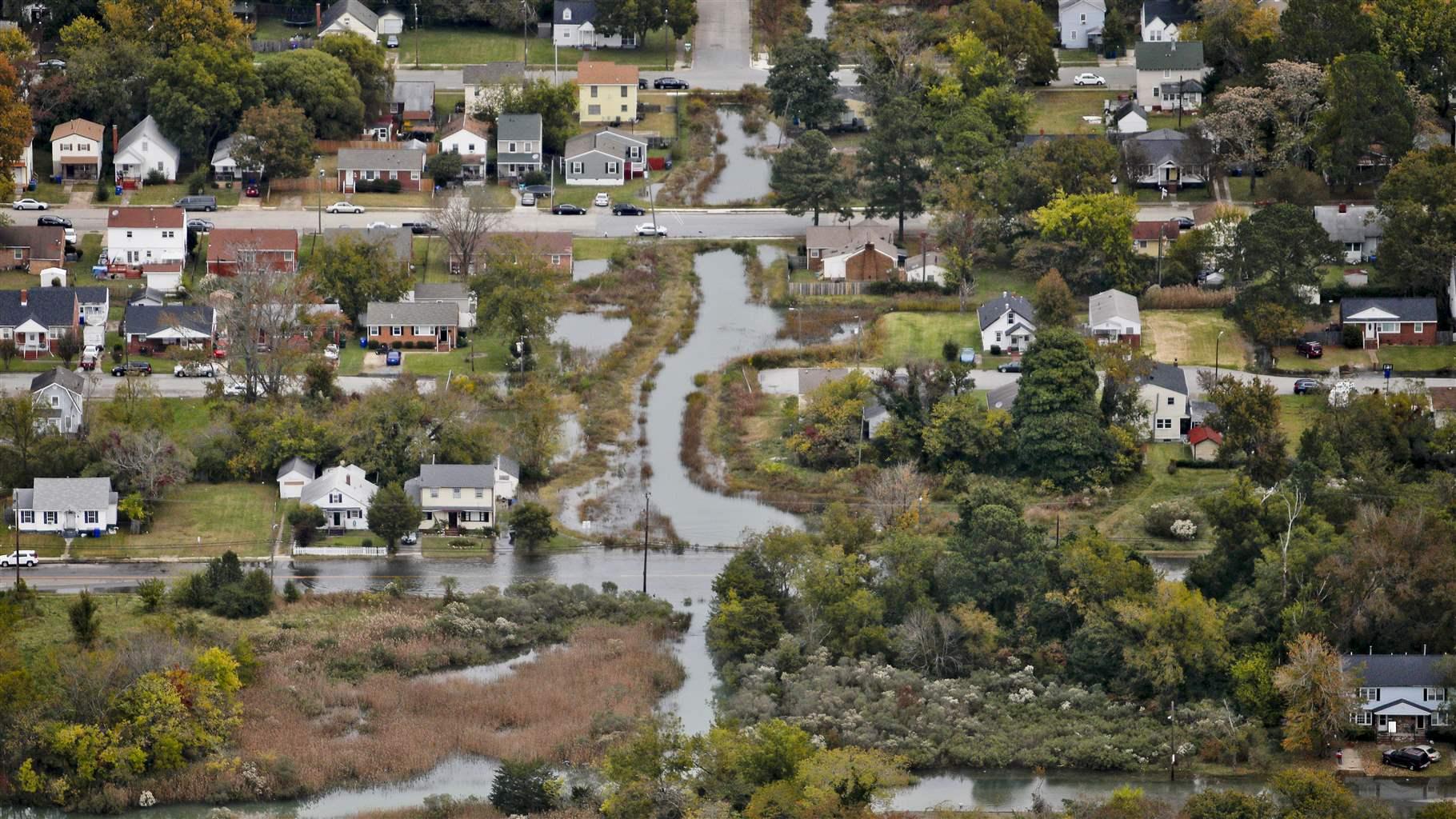This detailed aerial photograph showcases a suburban neighborhood abundant with trees and foliage, and a river that runs through it, featuring a picturesque bridge. The neighborhood comprises mainly residential, well-maintained, single-family homes, most of which are two stories, while a few are single-story. The homes near the river suggest that the area is ideal for nature enthusiasts. However, the image also reveals a concern; it appears that the neighborhood might be experiencing the onset of flooding. Water is visible on the streets, and it seems to be gradually posing a challenge for residents. Some cars are parked on the street, where the ground visibly looks wet. The situation isn't severe yet, but continued rainfall could potentially impede residents' ability to navigate their driveways, particularly evident with a house situated in the center of the image.